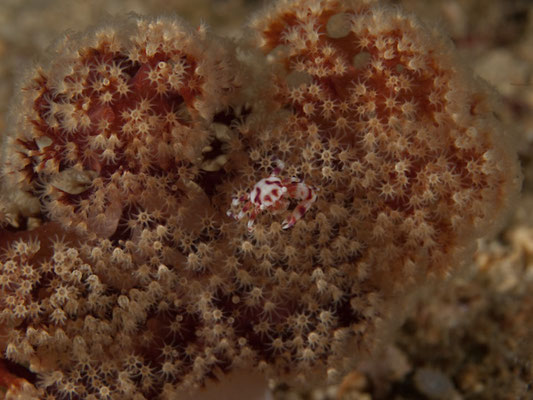In this underwater image, a small, predominantly white crab with striking red stripes is situated right in the center. Though taking up only about 10% of the frame, the crab is easily noticeable amidst its surroundings. The crab rests atop what appears to be a piece of coral, characterized by fluffy, flower-like structures that cover most of its surface. The coral itself exhibits a varied palette with its base being a dark, rusty brown while the light beige, fluffy extensions create a striking contrast. The background is mostly out of focus, with glimpses of the blurry seafloor adding depth to the scene. The overall ambiance suggests a dimly lit underwater environment, highlighting the natural camouflage abilities of the crab and the intricate details of the coral.